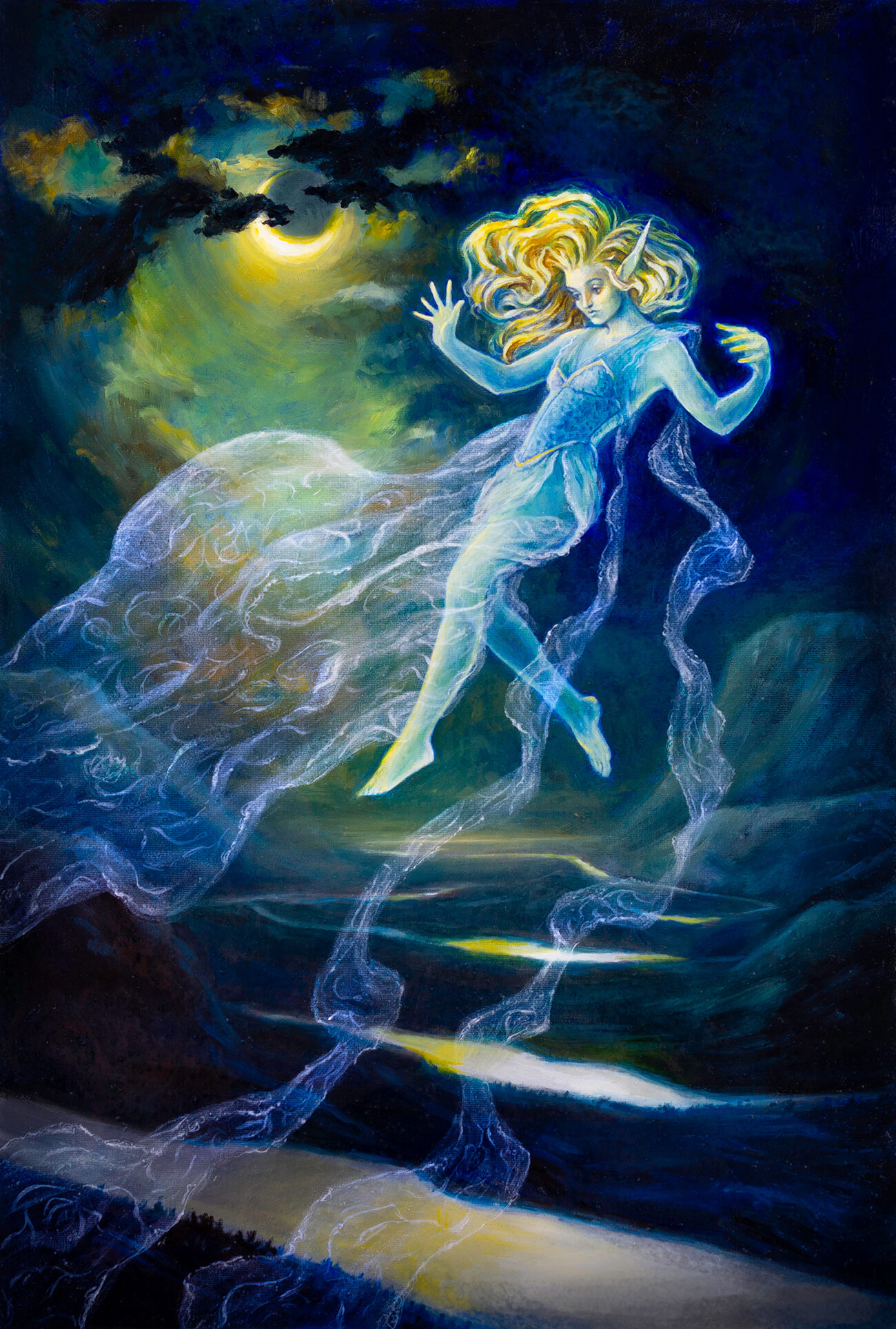The image is an ethereal fantasy painting set at night, dominated by blue hues with some accents of green and yellow. It depicts a floating female elf with long blonde hair that waves around her as if she is underwater. She has distinctly pointed ears and a semi-translucent, flowing blue dress that extends off the edges of the painting, accompanied by trailing spectral ribbons. The elf's body emits a glowing blue and white light, adding to her ghostly presence. Her arms are extended out to her sides, and her legs are positioned as if she is dancing mid-air. Behind her, a dark forest landscape is visible with a river flowing through it, and faint outlines of mountains in the distance. The sky features a crescent moon partially obscured by dark clouds, which casts a ghostly yellow and gray glow, creating a mystical atmosphere. The moon's mysterious light reflects off the lakes or pools of water below, enhancing the dreamlike quality of the scene.